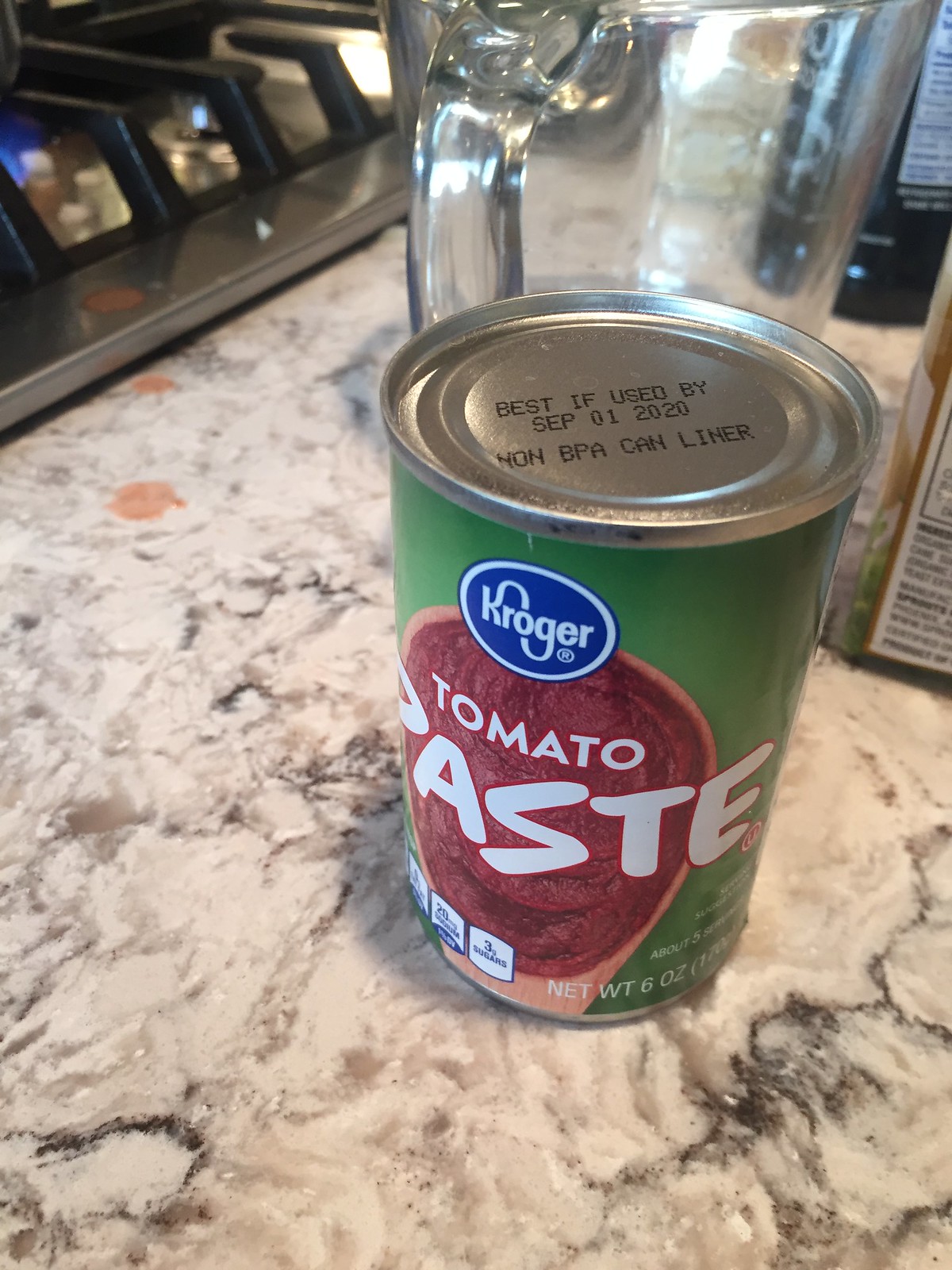The photograph captures a white marbled countertop with streaks of dark black and gray. At the center of this countertop sits an unopened can of Kroger tomato paste. This green-labeled can prominently features a brown spoon filled with tomato paste in the center. The label includes a blue oval at the top with the Kroger logo in white letters, and below, in larger white letters, it reads "tomato paste." The can's silver top displays text indicating it is best if used by September 1, 2020, and also notes that it has a non-BPA can liner. Behind the can, there's a clear glass pitcher or measuring cup, and to the left, part of a gas stove is visible. Additionally, on the right-hand side, there's a partially visible bottle or package with a bit of its white label showing. Some drips of a liquid are also noticeable on the countertop.